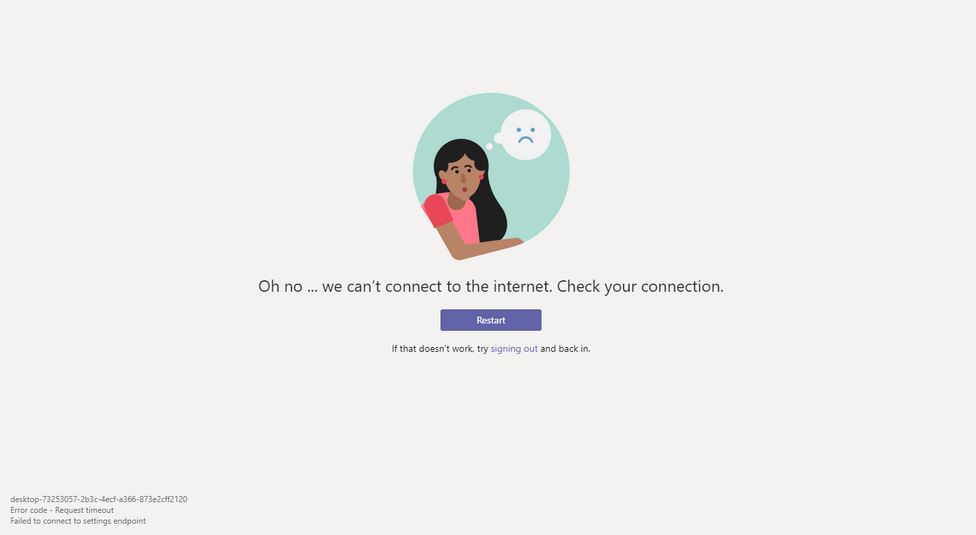The image features a tan background with a central circular graphic of a young Black girl. She has black hair and is wearing red earrings and a pink shirt with hot pink sleeves. Emerging from her head is a thought bubble containing a sad face emoticon and text that reads, "Oh no, we can't connect to the internet, check your connection." Below the message in the thought bubble is a purple box that says "Restart." Additionally, instructions are provided: "If that doesn't work, try signing out and back in," accompanied by a clickable purple icon for signing out. In the lower left corner, an error code displays "Failed to connect to settings." The upper portion of the image contains nondescript computer jargon. There is no branding or identifying information present anywhere on the image, giving it a generic and universal appearance.